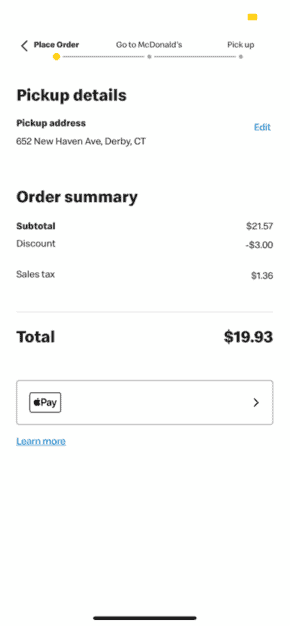This is an image of a smartphone or tablet screenshot depicting the ordering process for a food delivery app. The interface has a clean, all-white background with black text. At the top, there's a back arrow pointing left labeled "Place Order" in bold, with a yellow circle underneath, indicating the current stage of the process. A progress bar traverses the top, with dots marking the stages: "Go to McDonald's," and "Pickup." At the top right corner, a small yellow rectangle is present.

Below the progress bar, the section title "Pickup Details" is prominently shown in bold, followed by "Pickup Address" in smaller, bold font. The address listed is located in Derby, Connecticut, with a blue "Edit" button aligned to the far right. Below this, larger, bold text reads "Order Summary," detailing different charges: "subtotal," "discount," and "sales tax," each with corresponding amounts on the right side. A gray line separates these details from the final total, which is displayed in bold larger font, with “$19.93" aligned to the right.

At the bottom of the interface, there is a white rectangular button labeled "Pay" on the left side, accompanied by an image of an owl.